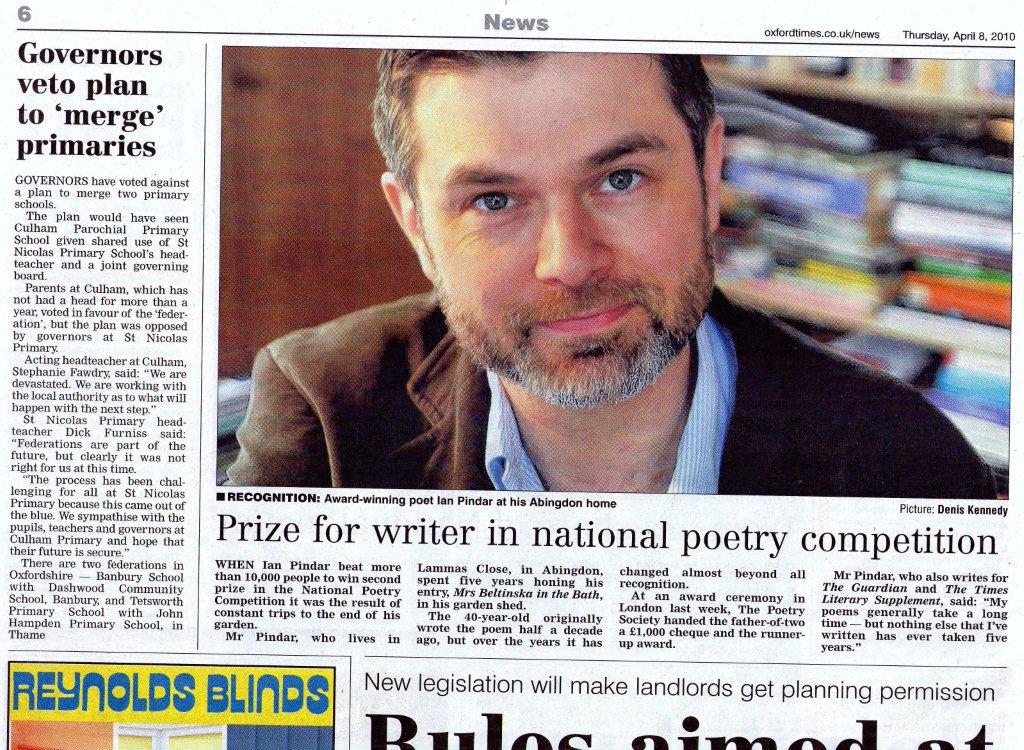This screenshot captures a segment of a newspaper page, meticulously laid out with various elements and articles. At the top center of the page, the word "News" is prominently displayed in a gray font, indicating the section of the newspaper. On the far left, the page number "6" is visible, and on the far right, the date "Thursday, April 8, 2010" is clearly marked.

Directly below these headings, a solid black line spans the width of the page, creating a visual separator. Beneath this line, a large, colored photograph of a bearded white male is prominently featured. He appears to be wearing a brown jacket over a blue shirt and looks directly at the camera.

The headline below his photograph reads, "Prize for Writer in National Poetry Competition," suggesting this feature article is celebrating his recent accomplishment. 

To the left of this main article, a different headline reads, "Governor's Veto Plan to Merge Primaries," indicating a political piece discussing a significant governmental decision.

In the bottom portion of the screenshot, the left corner displays the top part of an advertisement for Reynolds Blinds, with "Reynolds Blinds" prominently written in blue font against a yellow background.

To the right of this advertisement, the beginning of another news article is visible. The headline starts with "Legislation Will Make Landlords Get Planning Permission," hinting at new rules affecting property management. Additionally, the fragment below the headline reads "rules aimed at," suggesting the article's focus on regulatory changes.

Overall, the screenshot provides a detailed snapshot of the newspaper's page, featuring a mix of news articles, a prominent photograph, and advertisements.